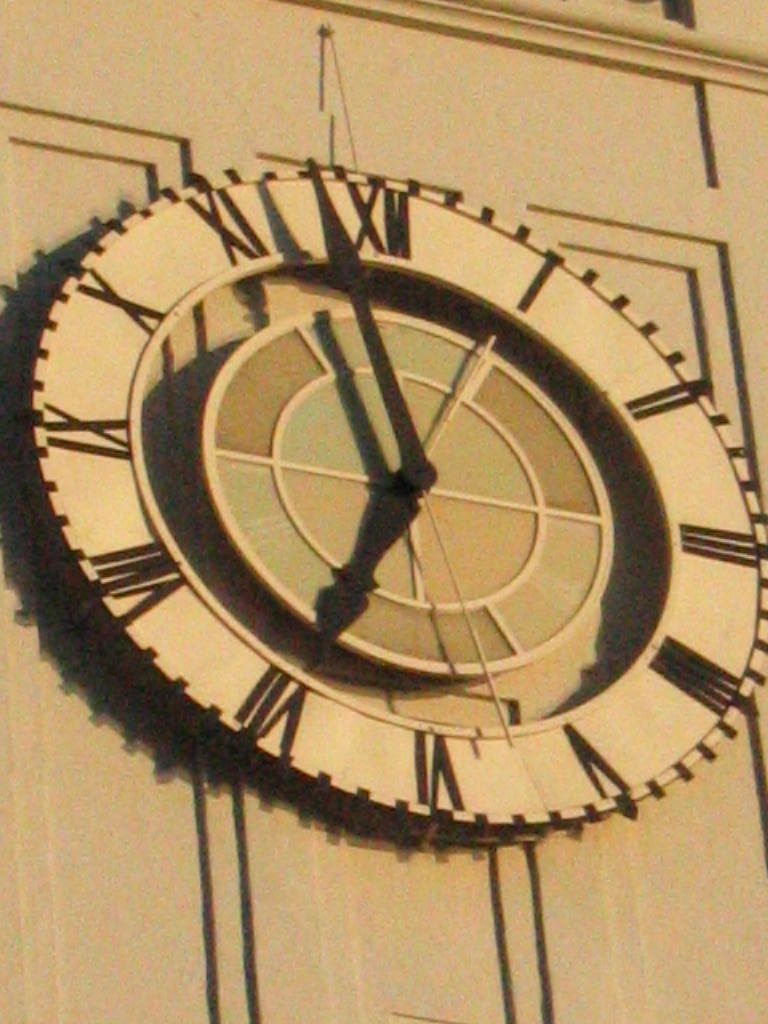This close-up photograph depicts a large clock mounted on an off-white or yellow-colored wall, possibly outdoors. The clock face displays Roman numerals from I to XII, with the thick, black arrow-shaped hour and minute hands indicating a time just shy of 7 o'clock, around 6:58. The clock is visually supported by a cable descending from above, which appears to secure the clock face against the wall. The wall itself features some design elements such as inlays and molding above the clock, adding to the architectural detail. The inner portion of the clock is adorned with a multicolored circular pattern reminiscent of a dartboard, consisting of segments in varying shades of green and yellow. The lighting creates a shadow cast to the left, suggesting a light source coming from the right. The image, while slightly blurry or filtered, appears professionally edited, enhancing the focus on the clock and the intricate details of its design and surroundings.